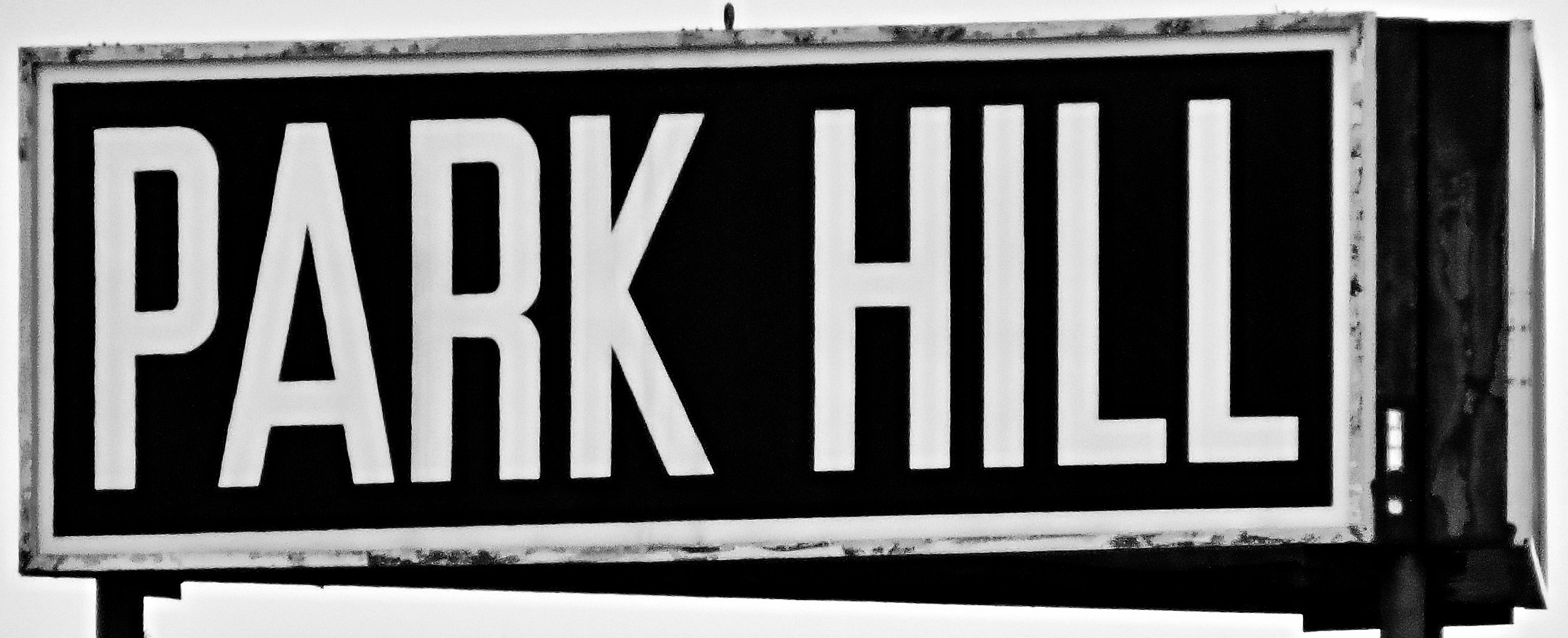This detailed, daytime photo captures a close-up view of a street sign for Park Hill. The image, taken from an angle that provides a three-dimensional perspective, showcases both the front and the side of the sign. Set against a backdrop of a clear daytime sky, the sign is rendered in black and white, characteristic of the signage in this area. A bold, dark background frames the words "Park Hill" in large, white, easily legible letters, bordered by a white outline. The sign exhibits visible signs of wear, with portions of the white border chipped and dirtied, suggesting it has been in place for a significant period.